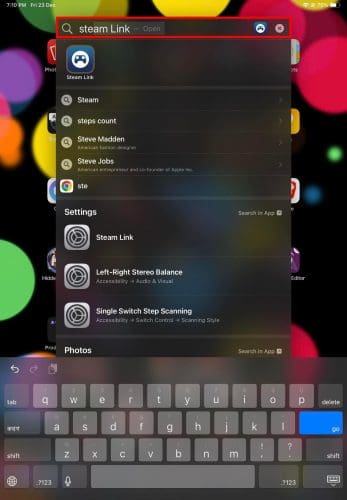The image is a screenshot taken from an electronic device that could be a computer, tablet, or phone, and features a wide display. The screen has a black background adorned with numerous circular lights of varying sizes and colors, including kelly green, yellow, red, purple, and orange. Some lights are large and vivid, while others are smaller but similarly colorful.

The screenshot contains a pop-up overlaying the background with icons partially visible behind it. At the top of the screen, status indicators can be seen but not clearly read; these include the current time, date (possibly Friday, the 23rd of December), internet connection status, and battery life, which seems to be in good condition.

The pop-up features an address bar with the text "Steam Link" and search results beneath it. These results include entries for "Steam," "Steam Count," "Steve Madden," "Steve Jobs," and various settings such as "Steam Link," "Left," "Right," and "Stereo Balance." At the bottom of the screen, a QWERTY keyboard is partially visible, indicating that text input is active. The overall composition of the screenshot is quite intricate and somewhat unusual.